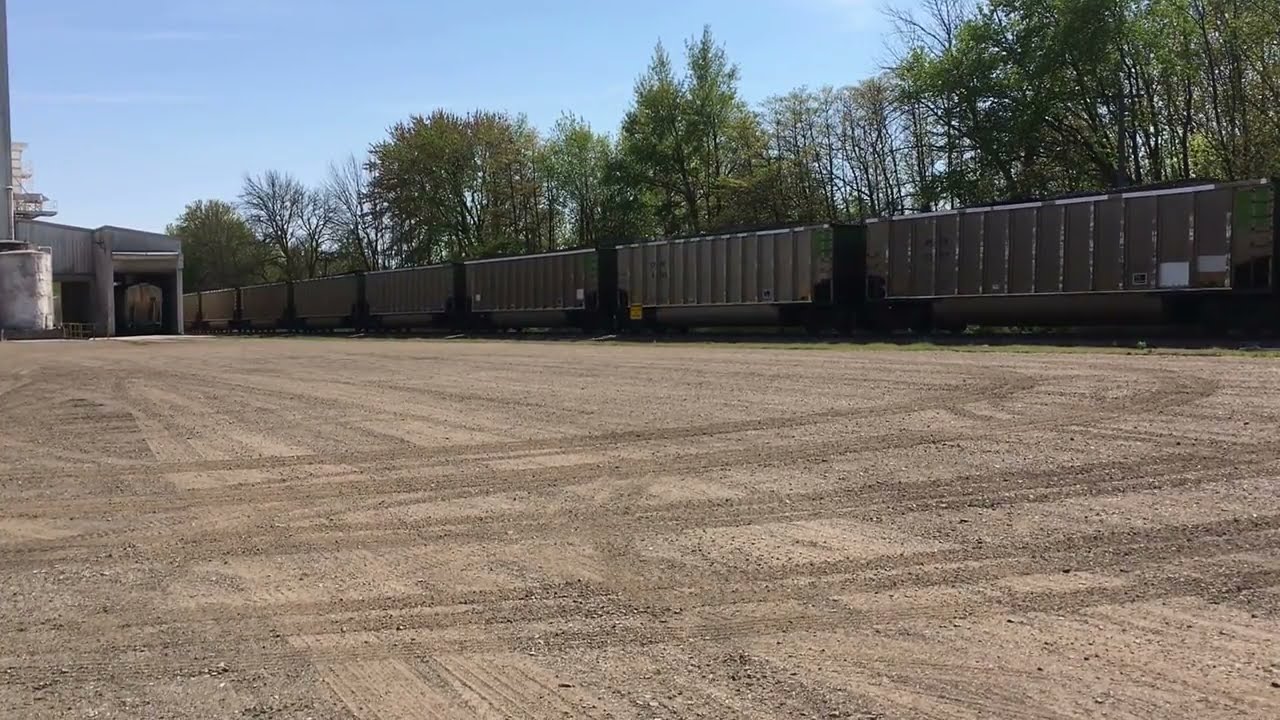This image depicts an expansive dirt or gravel lot, situated within an industrial area, possibly a train yard. In the foreground, the lot is clearly marked with tracks, suggesting the recent movement of vehicles. Dominating the right side and stretching towards the mid-left, there are several storage carts or train cars, totaling seven. These train cars are positioned near a line of lush green pine and maple trees, which form a dense forested backdrop. On the far left side of the image, partially obscured, there is a building that appears to be made of aluminum and includes a tall, white tank adjacent to it. The sky above is a pale blue, interspersed with a few flat, white clouds, indicating a clear, pleasant day. The overall scene is devoid of any people or active vehicles, reinforcing the industrial nature of the location.